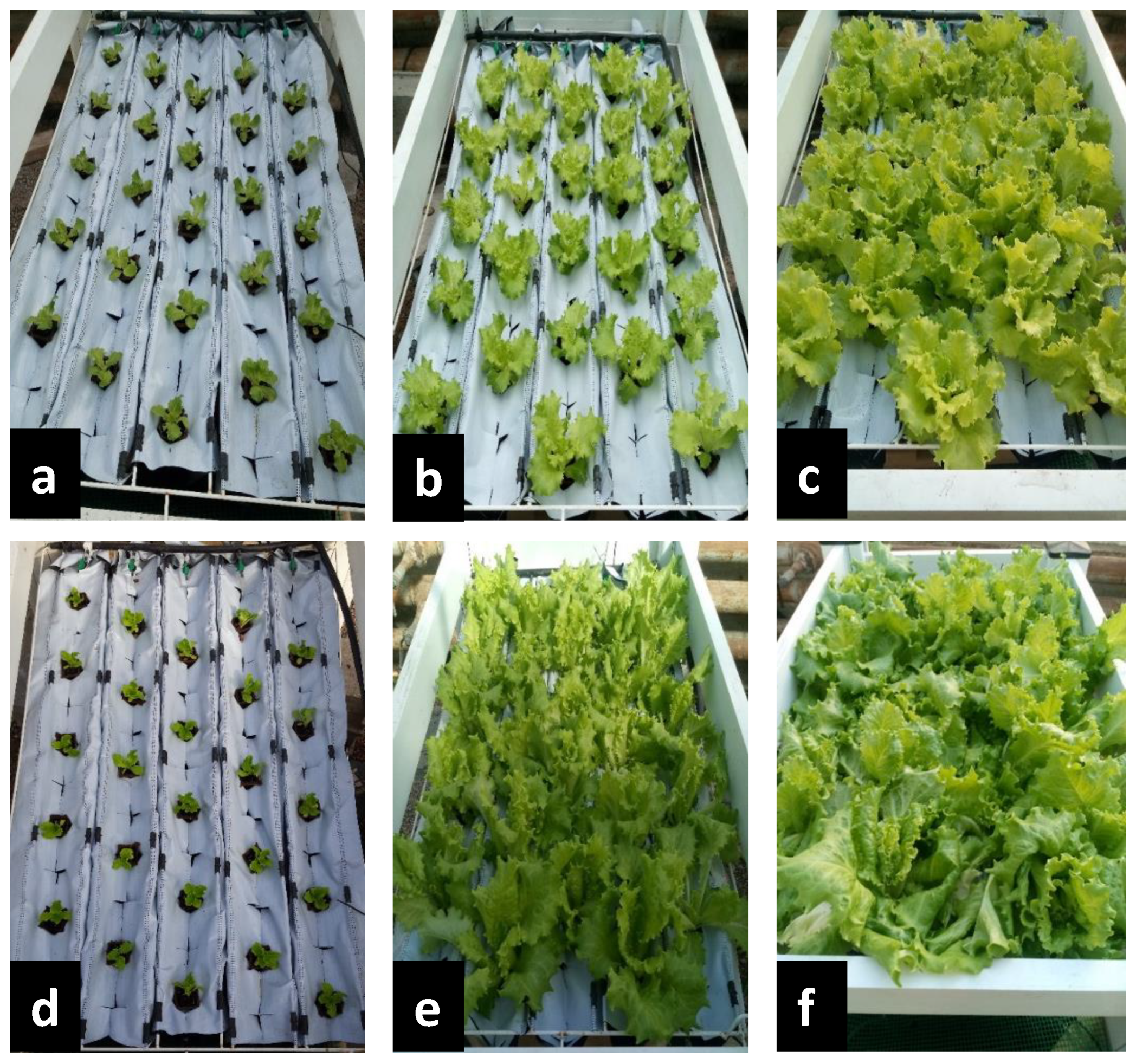The image is a detailed collage consisting of six vertically aligned rectangular pictures, separated by a thick white border. The top row features images labeled A, B, and C from left to right, while the bottom row includes images labeled D, E, and F. Each individual image displays the growth stages of lettuce, set against a backdrop of white plastic or fabric vertical strips laying flat.

In images A and D, the lettuce is shown in its initial, sparse stage with five vertical strips and scattered green leaves. As we move to images B and E, the lettuce has grown significantly, with the leaves appearing larger and more dense. By the time we reach images C and F, the greenery has become so abundant that it nearly obscures the white strips beneath.

The images collectively illustrate a time-lapse progression of lettuce growth, starting from small leaves to fully grown, lush patches. The setting is well-lit and clear, emphasizing the vibrant green of the lettuce against the stark white background.